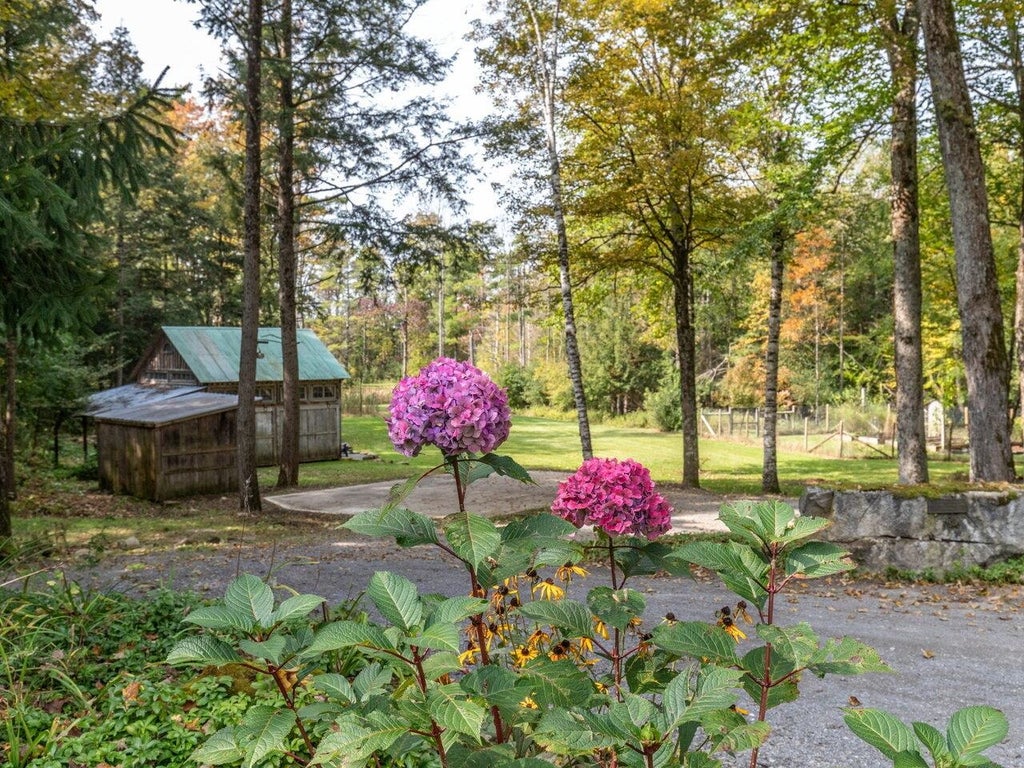This color photograph captures a picturesque nature scene featuring a small, aged wooden house or possibly a barn with a green roof, set in a beautifully wooded area. The bottom portion of the image showcases a flowering hydrangea bush with vibrant purple and fuchsia blooms, alongside cheerful black-eyed Susans with their bright yellow petals and dark brown centers. A gravel road leads up to the quaint building, framed by a mowed lawn. To the right, there is a fenced-in area that could serve as a garden or animal enclosure. Amidst the lush greenery, there are additional blooming flowers, including pink and yellow hues. The entire scene is bathed in sunlight, enhancing the serene and inviting atmosphere of this rural landscape, enveloped by a dense array of trees.